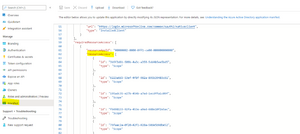The image depicts a blurry user interface page with unreadable tiny text against a white background. The main content comprises six distinct lines of bright blue text, each preceded by red text. On the far left side, there is a search bar above a vertical list of gray text items. Toward the bottom of this list, one word is highlighted in yellow. Additionally, the first line of the main blue text content is also highlighted in yellow.